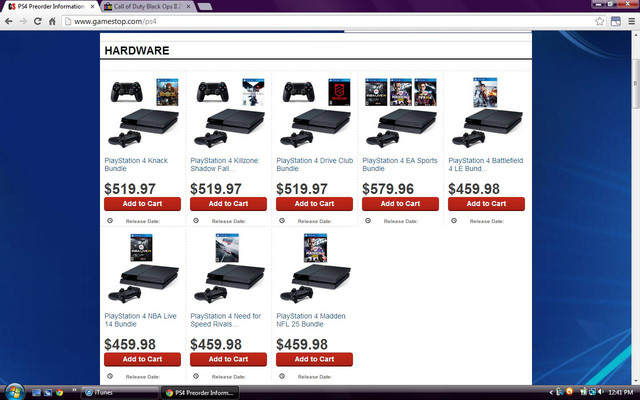This image depicts a webpage from GameStop's official website, specifically the section dedicated to PlayStation 4 hardware, as indicated by the URL 'GameStop.com/ps4' and the 'Hardware' label at the top left corner. The page showcases a selection of eight different PlayStation 4 bundles, with corresponding images and prices.

In the top row, the first three bundles are each priced at $519.97. The fourth bundle in this row is slightly more expensive at $579.96. The fifth bundle, which starts the bottom row, is priced at $459.98. Continuing along the bottom row, the prices of the next three bundles are $495.99, $459.98, and $459.98.

Each of these PlayStation 4 bundles includes specific games or additional content. The first bundle in the top row features a "Knack Bundle", while the last bundle in the bottom row is a "Madden NFL 25 Bundle". The website layout clearly indicates the various options available for purchase, helping potential buyers select the best bundle that fits their preferences and budget.